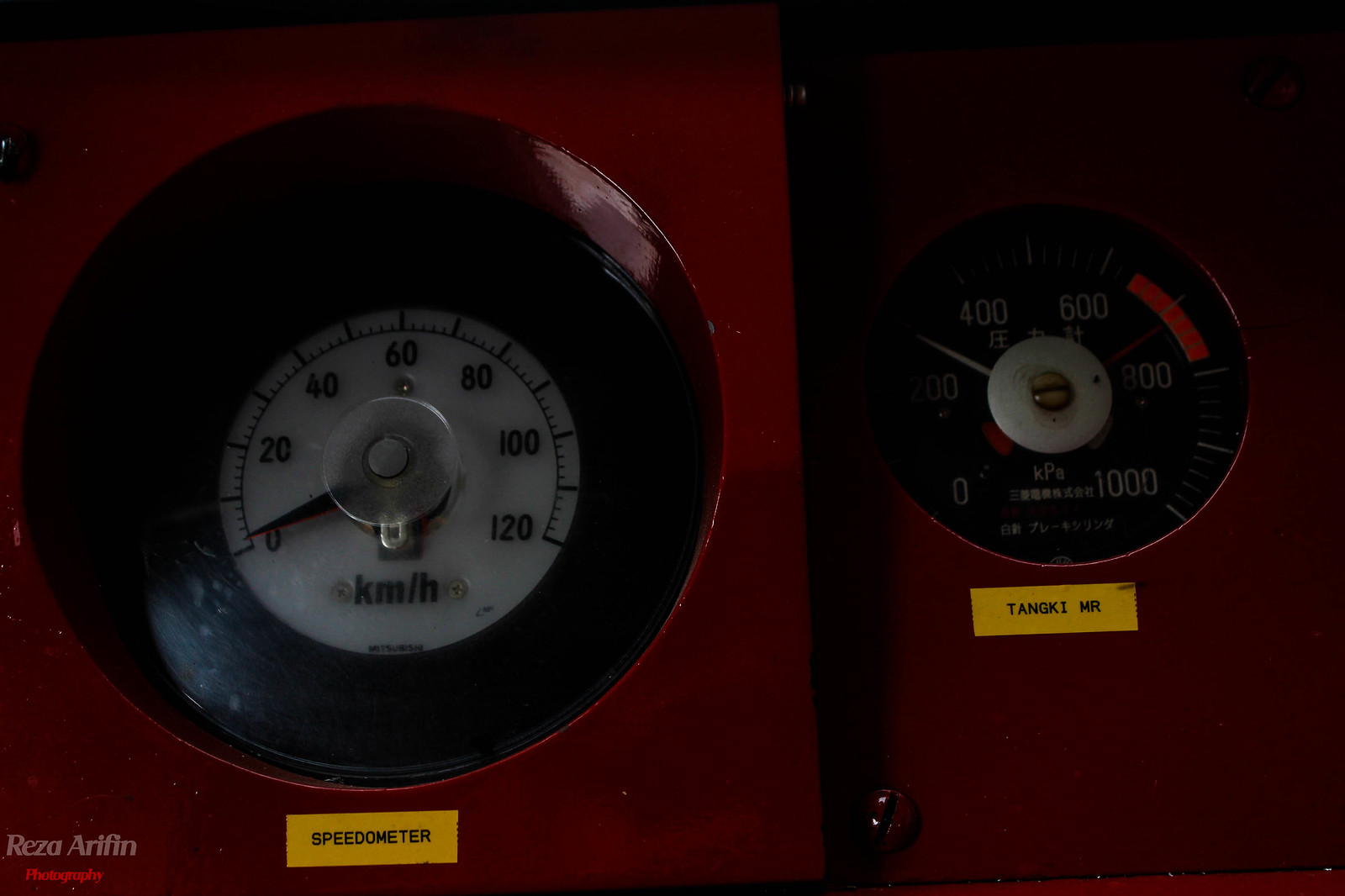In the image, there are two distinct types of control instruments, placed side by side, set against a red background. The left control is a circular speedometer with an orange label underneath that reads "speedometer" in black text. Further below in the lower left corner, there is white text displaying "Risa Ariflin," accompanied by some illegible bright red text underneath it. The circular speedometer has a black face with a white center, and it features a gauge and an arrow. The gauge increments in 10s but only displays numbers at intervals of 20 (0, 20, 40, 60), with intermediate lines marking the increments.

To the right, positioned slightly lower in depth, is another measuring instrument. This device also has a black background with white numbers, graduating in larger increments compared to the speedometer, showing values at 0, 200, 400, 600, 800, and 1000. At the center of this gauge, there is a white section labeled "TANGK1MR." The contrast in placement and detail suggests that both controls belong to either an old car or another piece of equipment, although they serve different functions.